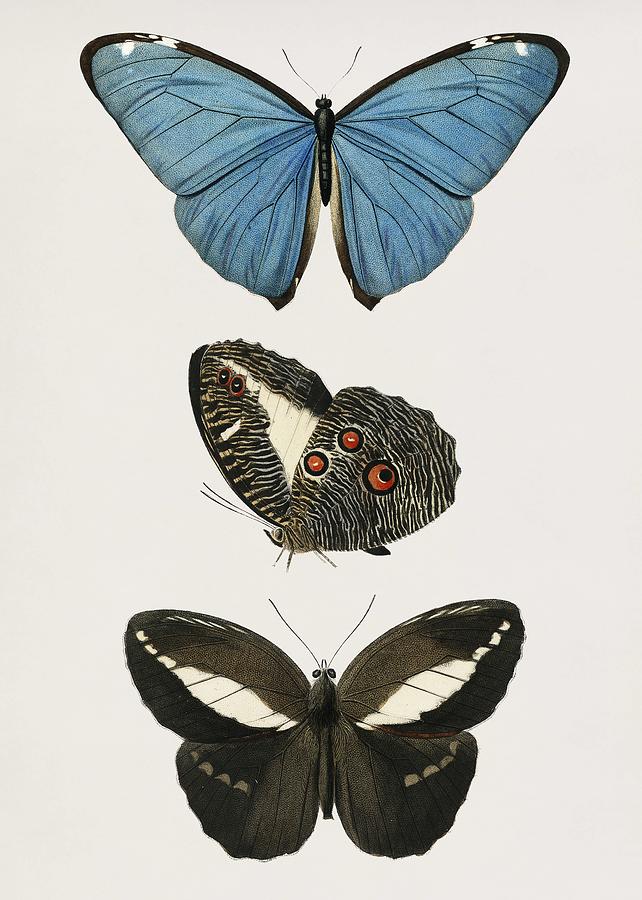This botanical illustration, portrayed in a vertical, portrait orientation on a very light pink background, features three distinct and carefully detailed butterflies. The first butterfly at the top showcases striking blue wings with subtle white tips, delicately outlined in black, and intricate light black veins coursing through both the upper and lower sections of the wings. Its small body and antennae are prominently positioned between the fully spread wings. 

Below it, there is a moth, depicted in profile as it faces the left side of the image. Its wing, facing the viewer, is adorned with three brass-colored, eye-like markings near the top center, set against a backdrop of black and white striped patterns.

The bottom butterfly in the illustration is predominantly black with distinctive white patches at the center of its wings and white dots toward the wing tips. Its intricate black body is slender, and it also features noticeable antennae. All three insects are meticulously aligned from top to bottom, highlighting the rich detailing and precision typical of botanical illustration art.